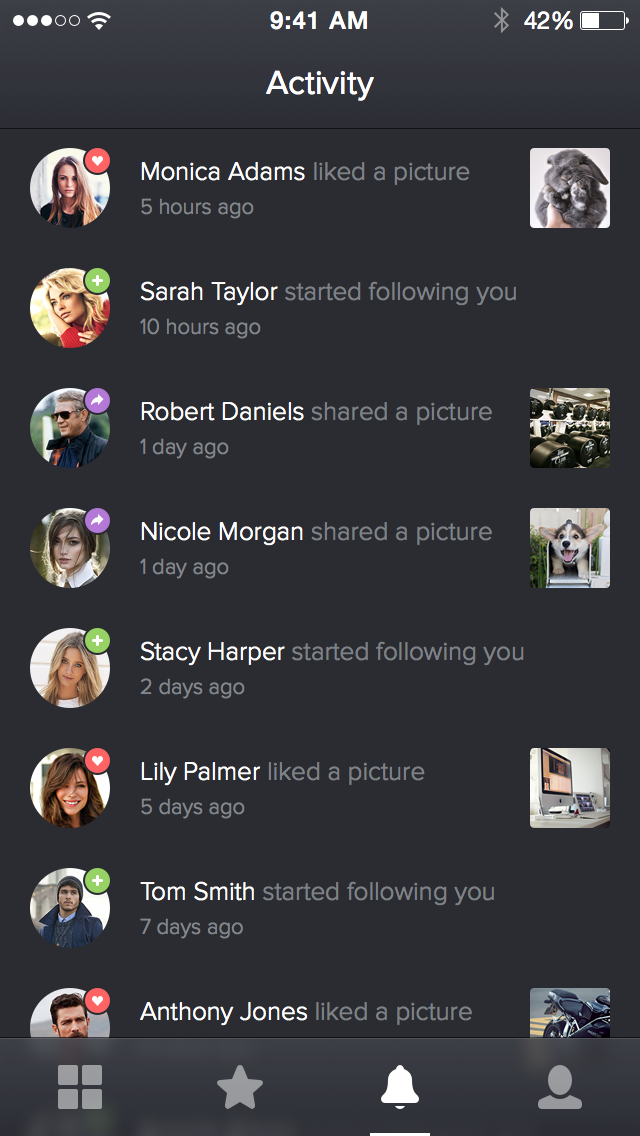This is a screenshot of the activity page on a social media app, displayed on an iPhone. The background color is a dark gray, providing a sleek and modern aesthetic. 

The top of the page shows the heading "Activity Invite." Below this, the left side of the screen features various user's profile pictures in circular icons. Each icon is accompanied by notifications detailing recent interactions: Monica Adams liked a picture, Sarah Taylor started following you, Robert Daniels shared a picture, Nicole Morgan shared a picture, Stacey Harper started following you, Lily Palmer liked a picture, Tom Smith started following you, and Anthony Jones liked a picture.

At the bottom of the screen, four icons are prominently displayed. From right to left, these include a user or account settings icon, an activity icon shaped like a bell, a star icon, and a four-tile icon which presumably navigates to the main page of the app. This well-organized interface allows the user to easily stay updated on their social interactions and manage their account settings efficiently.